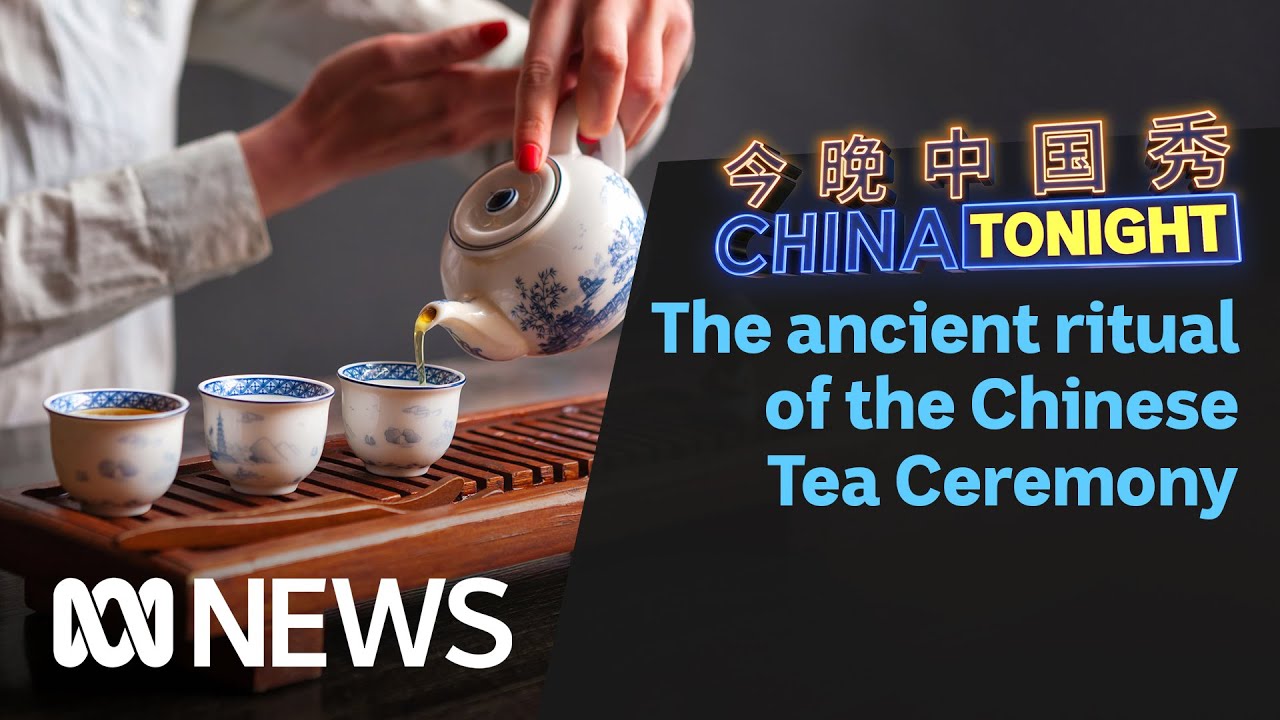In this advertisement image, set against a black background, the right side features text with Chinese characters at the top, followed by "China Tonight" where "China" is in bright blue and "Tonight" in a yellow box. Below, in lighter blue, it reads "The Ancient Ritual of the Chinese Tea Ceremony." On the left side of the image, a close-up photograph captures a woman, distinguishable by her polished red fingernails, wearing a white shirt. She is meticulously pouring tea from a blue and white teapot into three matching cups placed on a wooden board with slits for spills. Below this scene, a logo resembling a DNA swirl and the word "NEWS" in bold white letters are prominently displayed, indicating that this is an advertisement to watch the traditional tea ceremony on television.